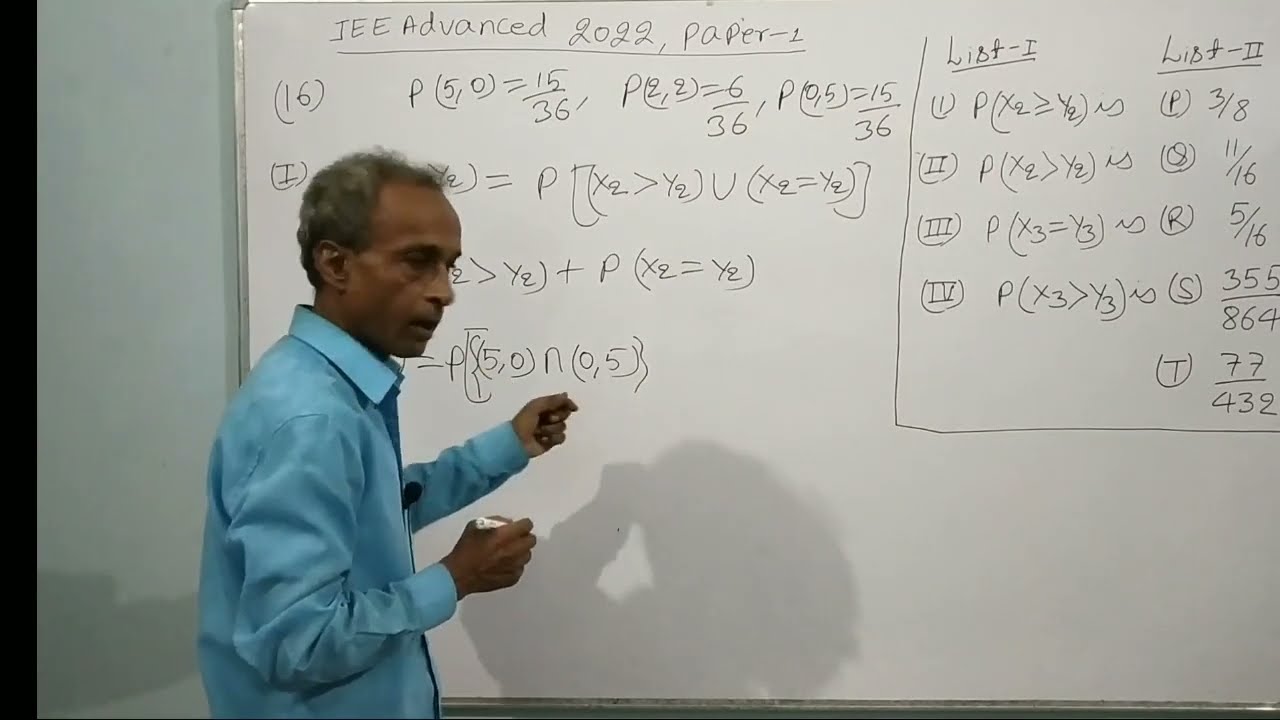The horizontal rectangular photograph captures an older man, potentially a teacher or analyst, standing by a large whiteboard covered with intricate writing. He is holding a marker in his right hand and gesturing towards the board with his left. He has short, salt-and-pepper hair and darker skin, and is dressed in a long-sleeve, collared blue button-down shirt. The whiteboard features extensive mathematical notations, including fractions, problem number 16, and two columns labeled "list-1" and "list-2." At the top, it reads "JEE Advanced 2022 Paper-1." The wall adjacent to the whiteboard is a very light mint or bluish color. The man is slightly blurry and some of his shadow is visible on the whiteboard and the wall behind him, suggesting he is engaged in explaining or discussing the content on the board.